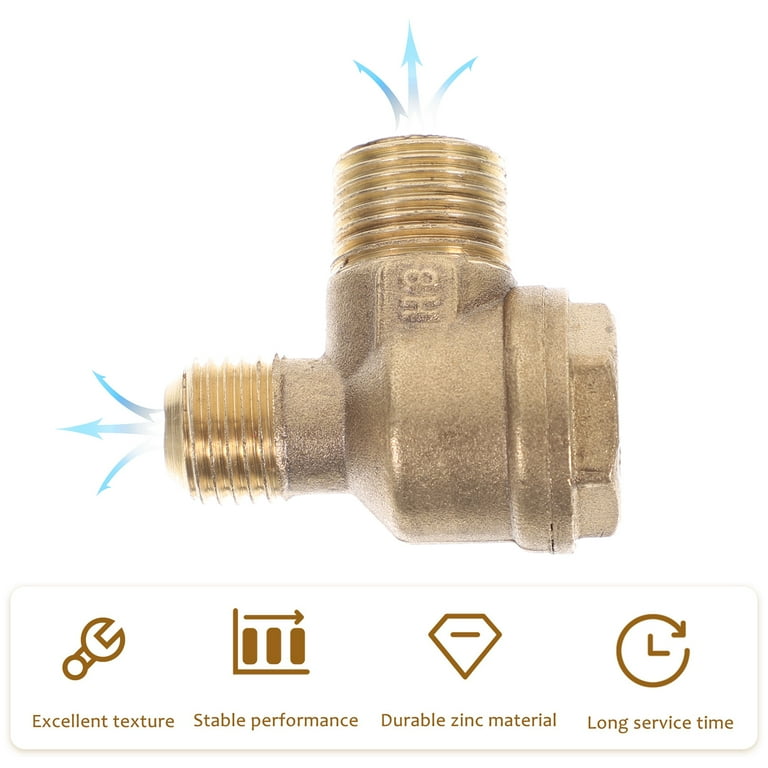This image depicts a brass plumbing component designed for diverting the flow of water or gas in a piping system. The device features multiple threaded outlets: a larger input on the right, a medium-sized output on the top, and a smaller output to the left, forming right angles. An imprint on the device reads "H8," though it could also be interpreted as "8H," depending on orientation. Below this marking, there's a panel featuring several icons and text: a wrench icon with the words "excellent texture," an unclear icon with "stable performance," a diamond-shaped icon indicating "durable zinc material," and a clock icon stating "long service time." Arrows illustrate the flow direction, further emphasizing the piece's function as a routing or reduction device within a plumbing system. Despite the mention of zinc in the text, the component’s brass material is evident from its color.